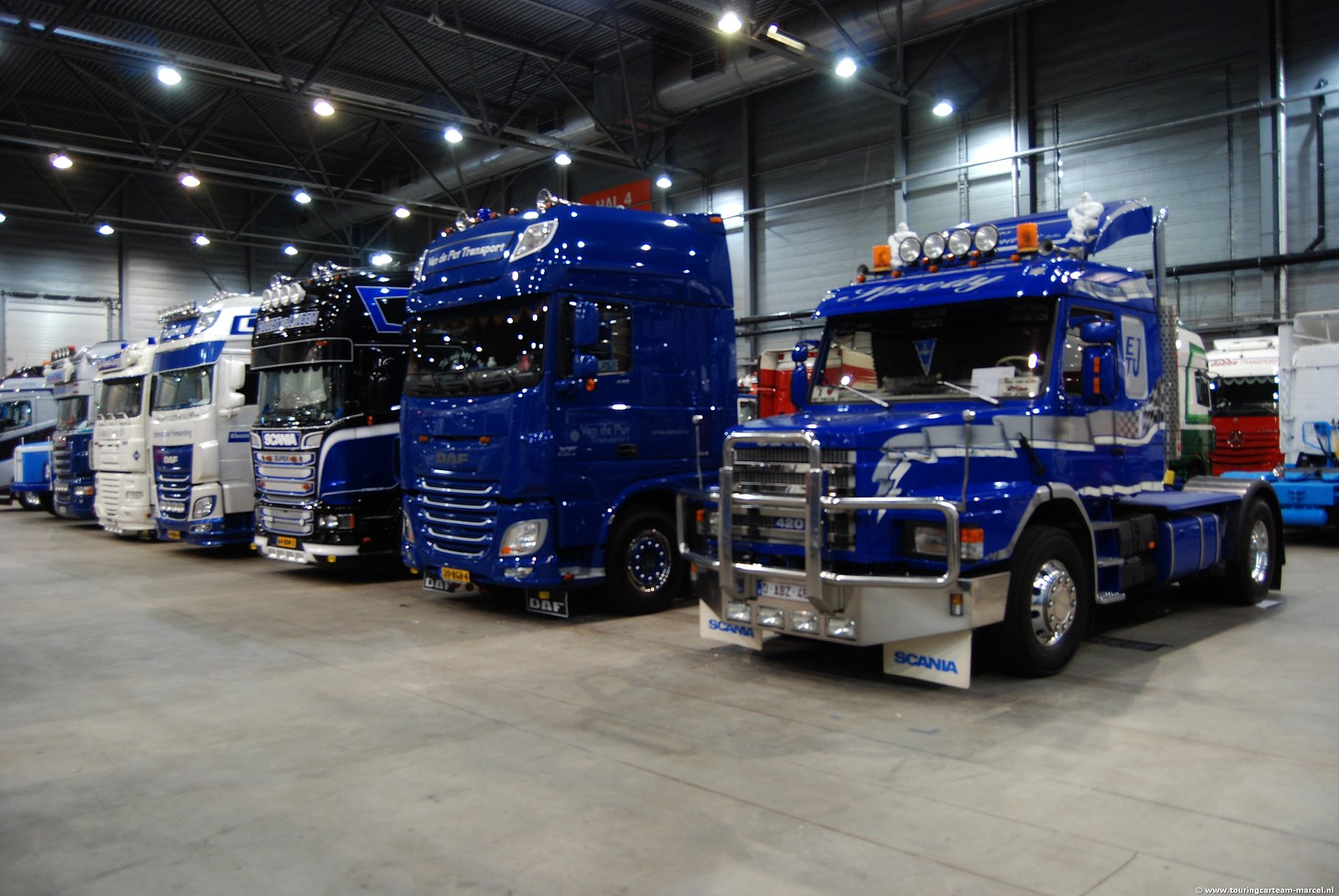This color photograph captures the gleaming front cabs of numerous semi-trucks neatly arranged inside a spacious, industrial-style warehouse. The warehouse features a spotless, slate-gray cement floor and a blue-gray metal back wall, which adds to its modern, industrial aesthetic. Beams and circular hanging lights illuminate the scene, accentuating the shiny, seemingly brand-new paint jobs on the trucks.

In the foreground, there are six or seven semi-truck cabs, displaying an array of colors: the first two are a bright blue, followed by a third in a striking combination of black and blue with white stripes reminiscent of a checkered flag. Two more trucks are solid white, and a few others in varying shades of blue and white can be seen in the background. Additionally, a red vehicle is partially visible towards the rear of the image, adding a pop of color. Black pipes along the walls further enhance the industrial feel of the space.